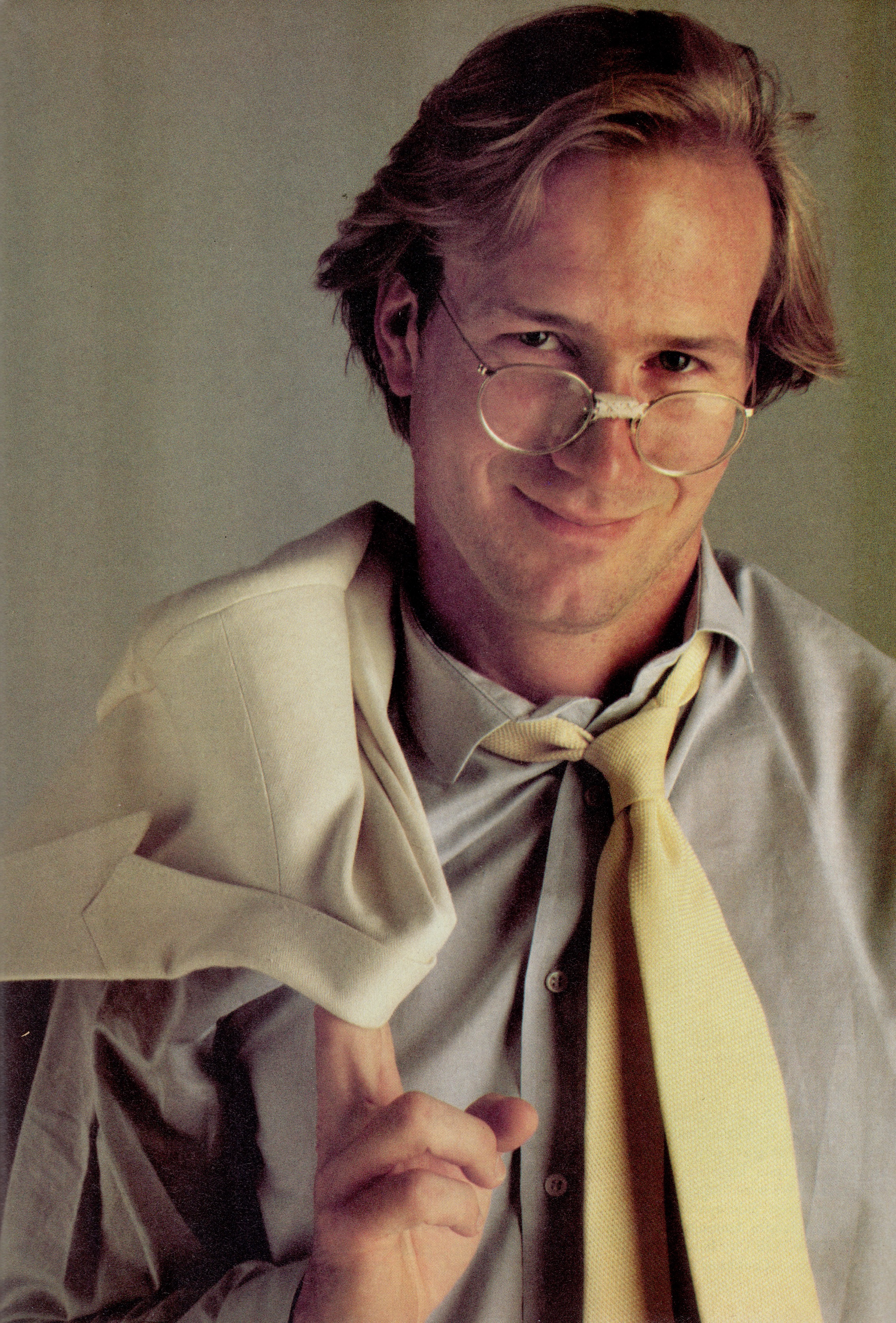A man with medium-length blonde hair and light brown eyebrows is smiling at the camera. He wears thinly clear-rimmed glasses, which have a piece of tape in the middle suggesting they were broken. He has on a grey shirt, buttoned up except for the top button, with light grey buttons. Around his neck, a yellow necktie hangs askew, with both pieces visible. Over his right shoulder, he drapes a light cream-colored blazer, hooked onto his first and second fingers. The background is a light grey shade, closely matching his shirt. His overall appearance is somewhat reminiscent of William Hurt.